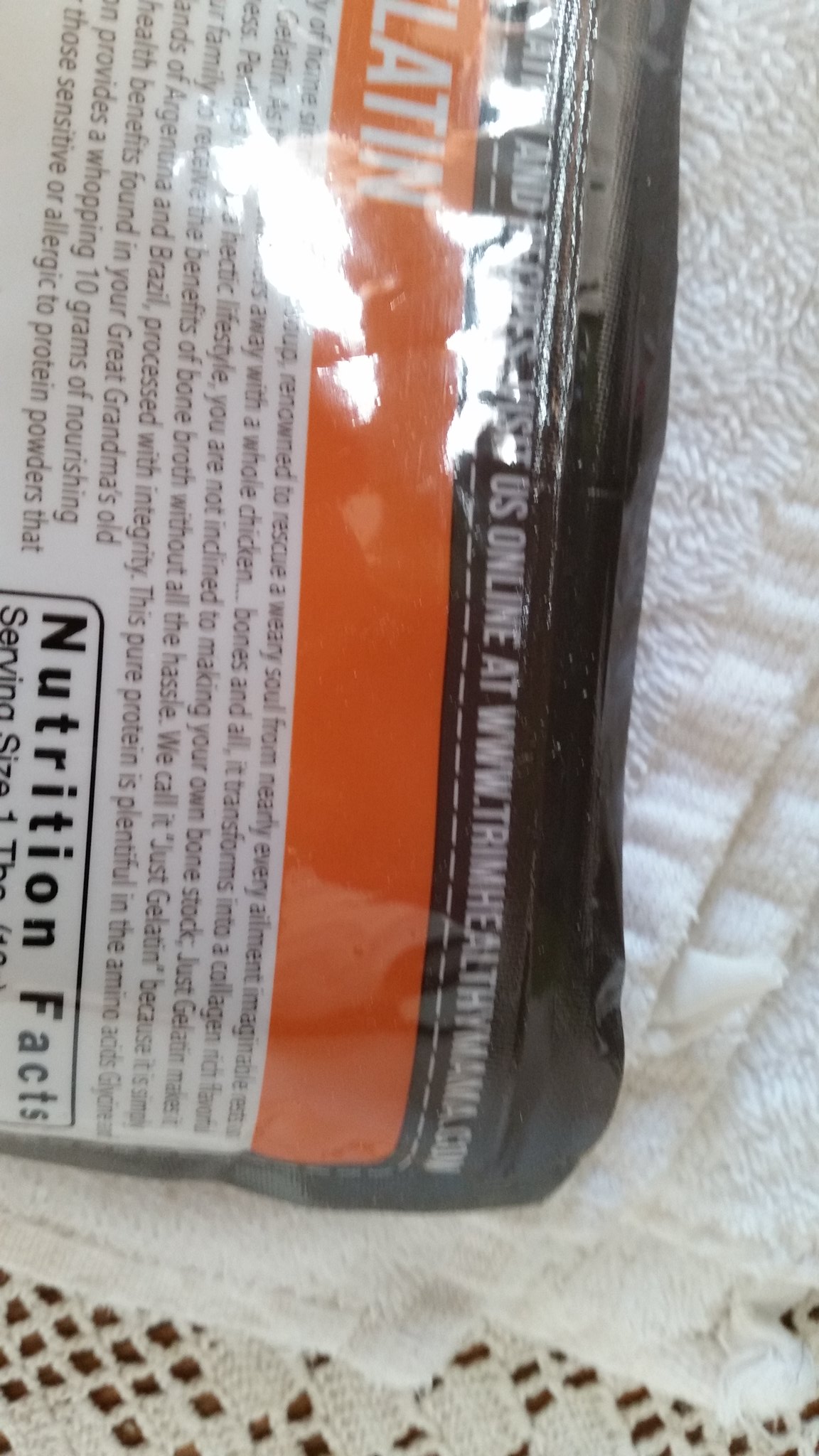This image features a close-up shot of a food package resting on a folded white towel placed atop a delicate doily, all set on a rich brown wooden table. The plastic packaging is glossy, with light reflecting off its surface and creating a subtle glare. The photograph captures the back of the package. The top section of the package is brown, followed by an orange label with the word "Latin" prominently displayed in white letters. Below this, the label turns white with dark brown lettering, indicating a detailed description of the product. In the bottom right corner, the nutrition facts are clearly visible, enclosed within a simple black border.